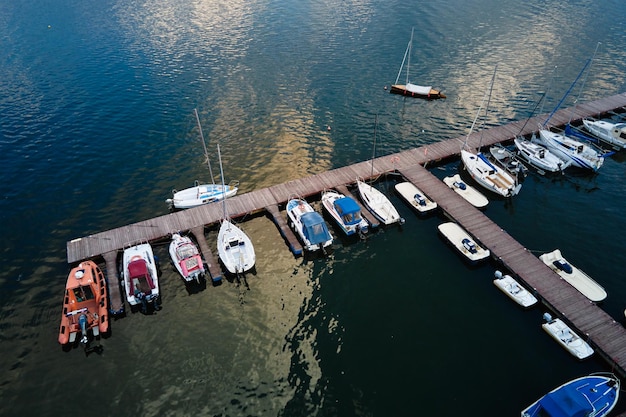This aerial, horizontal, rectangular photograph captures a sprawling T-shaped boat dock at what appears to be a marina, surrounded by dark-colored water with patches of floating mud. The dock features a long central pier leading out to the crossbar of the 'T,' providing ample spots for various types of boats, including speedboats, motorboats, fishing boats, and rowing boats, as well as sailboats with sails down. Every sleeve of the dock is occupied, with an array of primarily white vessels, but also a distinct blue boat and a singular orange boat that stands out, evoking the image of a fire truck. Notably, a sailboat rests at the very base of the central bar, and another one is moored on the other side. Additionally, two boats are intriguingly positioned outside the main docking area. This serene daytime scene captures the calm, intricate layout of the marina, with boats neatly arranged against the tranquil backdrop of the water.